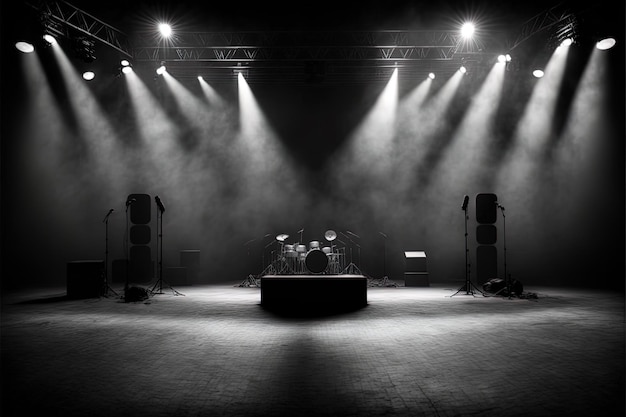This black and white photograph captures an evocative scene within a studio, characterized by its raw, industrious atmosphere. The wooden paneled floor extends across the space, holding an array of musical equipment bathed in stark lighting. Overhead, metal scaffolding supports intense, white studio lights, creating dramatic shadows and illuminating fog that lends a smoky ambiance throughout the setting. 

Central to the composition is a drum set, complete with visible cymbals, floor tom, bass drum, and kick drum, set against the background of other musical apparatus. Microphones stand poised around the drums, with two to three on either side, accompanied by several amplifiers and speaker towers situated in the distance. The entire scene, devoid of color, accentuates the silhouetted forms of the instruments and enhances the moody, concert-like atmosphere of the space. This meticulously lit and staged scene conveys the tension and anticipation before a musical performance, set on a seamless floor that blends the stage with the rest of the studio.